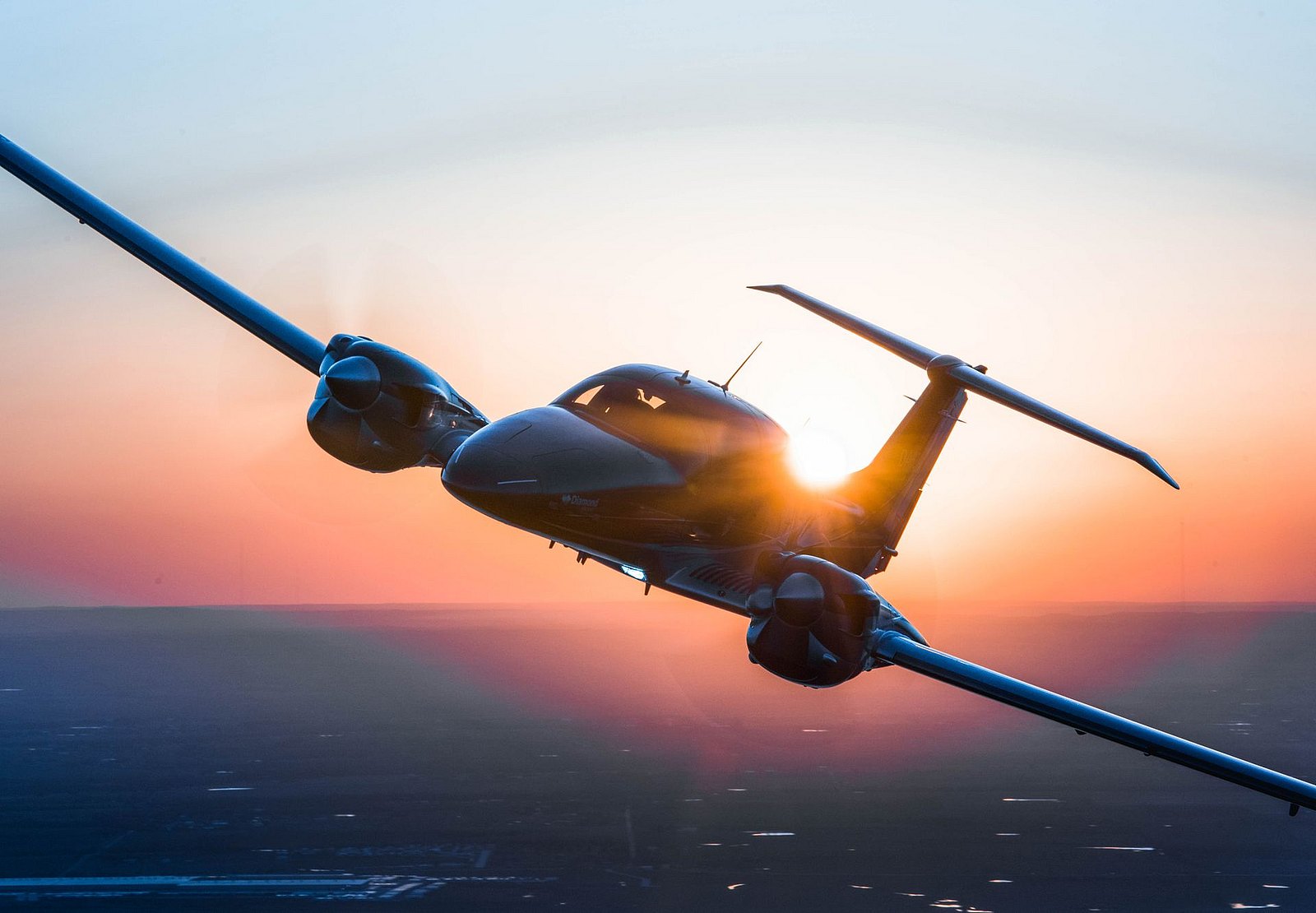This professional, full-color, outdoor photograph, taken during natural daylight, captures a small, twin-engine propeller plane mid-flight over a vast expanse of water. The square image features a serene sky transitioning from a light blue at the top to a warm reddish-orange near the horizon, indicative of an enchanting sunrise or sunset. The water below mirrors the sky's gradient and is marked with a few delicate, white-capped waves. The horizon line is evident just above the lower frame, enhancing the visual separation between the sky and sea. The focal point, the airplane, is positioned almost centrally, flying at a slight angle with one wing dipping towards the lower right corner and the other towards the upper left. This dark-colored plane, likely suitable for just a pilot and passenger, showcases its aerodynamic design with visible wings, motors, and a horizontal tailbar. The sun, partially obscured, glows between the cabin and the tail, casting a soft, golden illumination that adds to the overall warmth and tranquility of the scene.